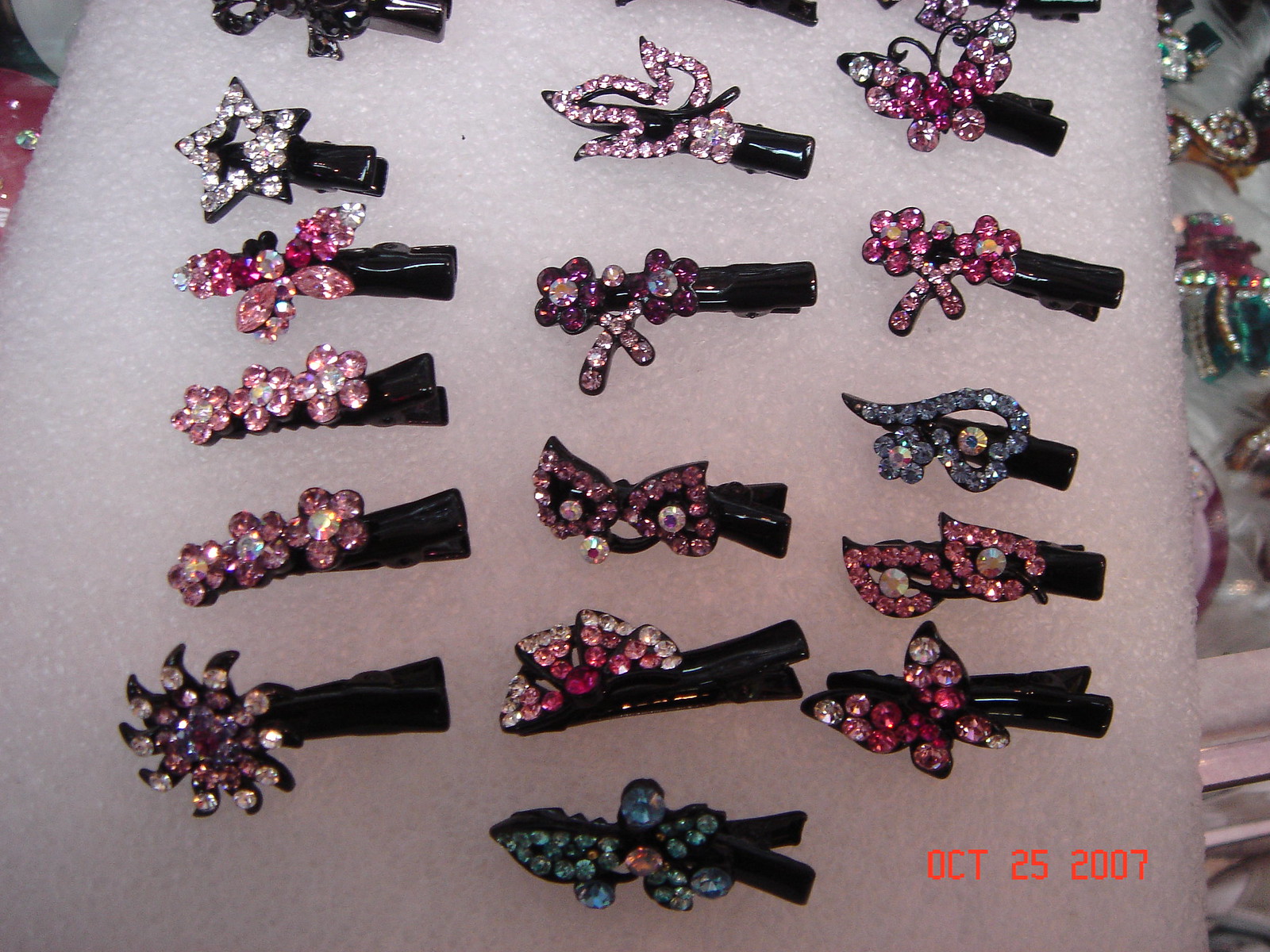The image dated October 25, 2007, captures a meticulously arranged display of costume jewelry, likely hair clips or brooches, set against a white background. The pieces are glittery, designed to mimic diamonds, and come in a variety of colors and shapes, including butterflies, flowers, and stars. Specifically, there are 15 visible pieces: some pink, purple, white, blue, or red, embellished with fake or rhinestone gems. Each piece seems to be fixed onto the white surface, which is described variably as styrofoam or velvet. The background of the image suggests that the display board is part of a larger collection, as more jewelry is visible beneath the main layer, hinting at a jeweler's personal collection or a retail display case. The time stamp in the bottom right corner confirms the date of the photo as October 25, 2007.